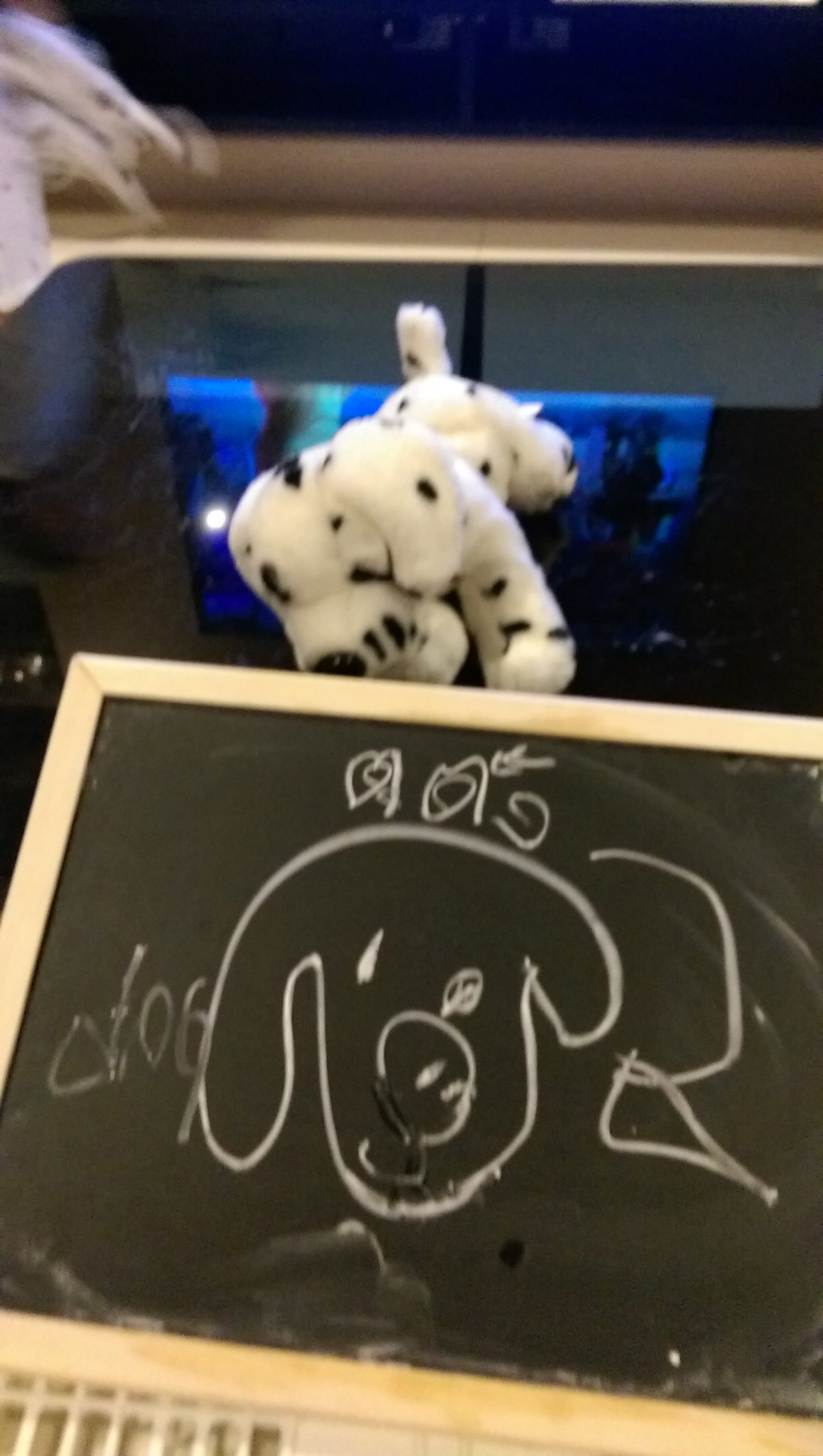This photograph features a wooden-framed chalkboard with a child-like drawing of a dog's face in the center. The chalkboard displays the word "dog" in lowercase letters to the left of the simplistic dog illustration, which includes round eyes, a nose, a mouth, and two drooping ears. There are curlicue squiggles above the dog’s head, and a vague D-shaped figure to the right that might represent the dog’s body. Below this chalk drawing sits a small, white stuffed Dalmatian with sparse black spots—one on its ear, three on its front legs, and a few on its face. The stuffed animal is positioned in such a way that it suggests the child was drawing it. The entire setup is placed on an indistinct blue square object and alongside some unidentifiable objects and a blurry backdrop. Elements within the scene hint at a possible laptop or LCD screen, but specific contextual details remain unclear.